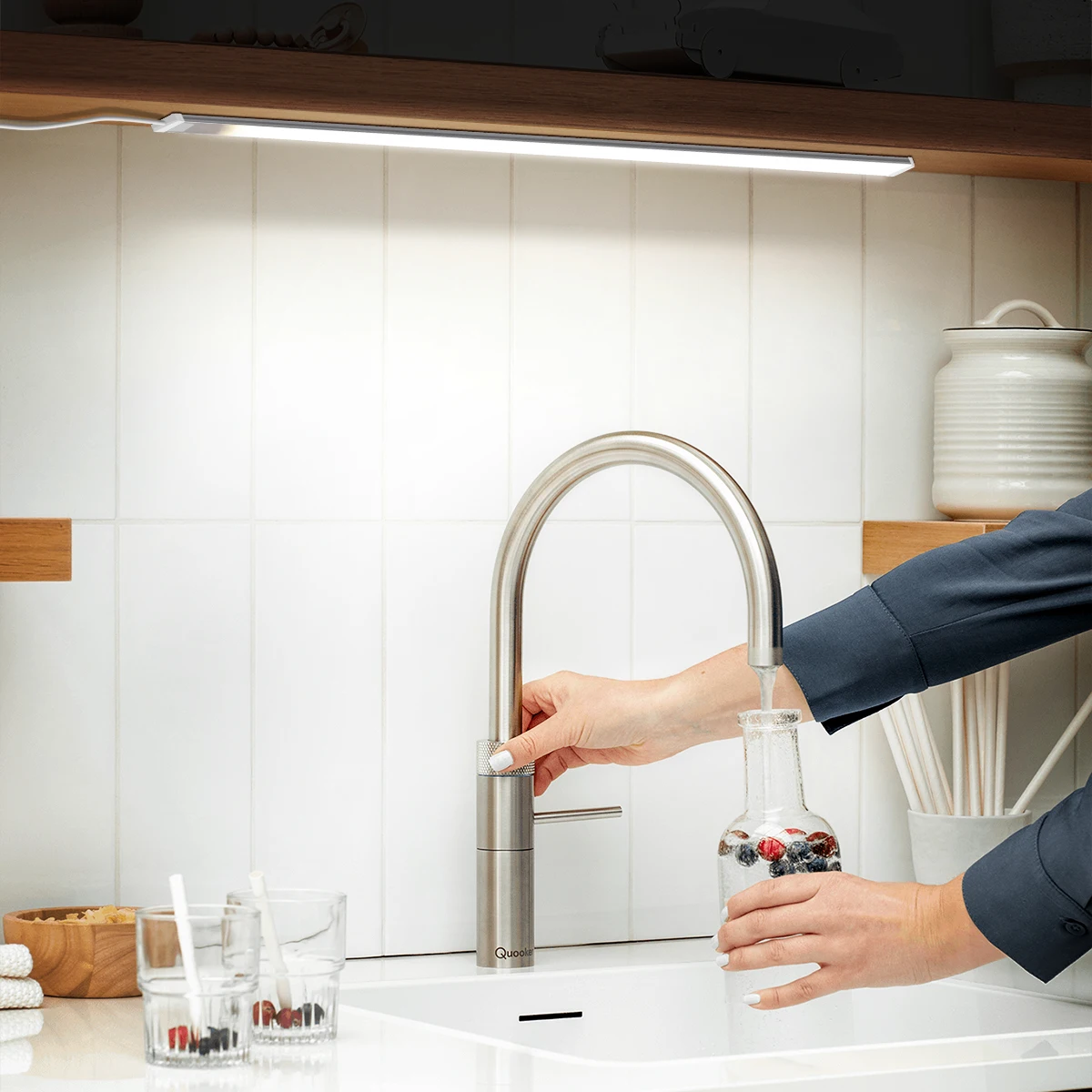The photo depicts a modern indoor kitchen with a focus on a sleek, silver stainless steel sink against a backdrop of pristine white subway tile backsplash. Overhead, an LED light attached to the upper cabinet illuminates the scene. A woman with black long sleeves is in the process of filling a clear, small vase-like glass with water from the touch-activated faucet. Inside the glass are blueberries and red berries, possibly raspberries. The flowing water sparkles as it pours in. To the left of the sink are two glasses containing a mix of strawberries or raspberries and blueberries, each accompanied by a white straw. Behind these glasses, a wooden bowl and white towel are also visible. The countertop is a clean, bright white, complementing the overall fresh and modern aesthetic of the kitchen. Floating shelves flanking the sink hold additional items, including white clay pots on one side and neatly folded dish towels on the other.